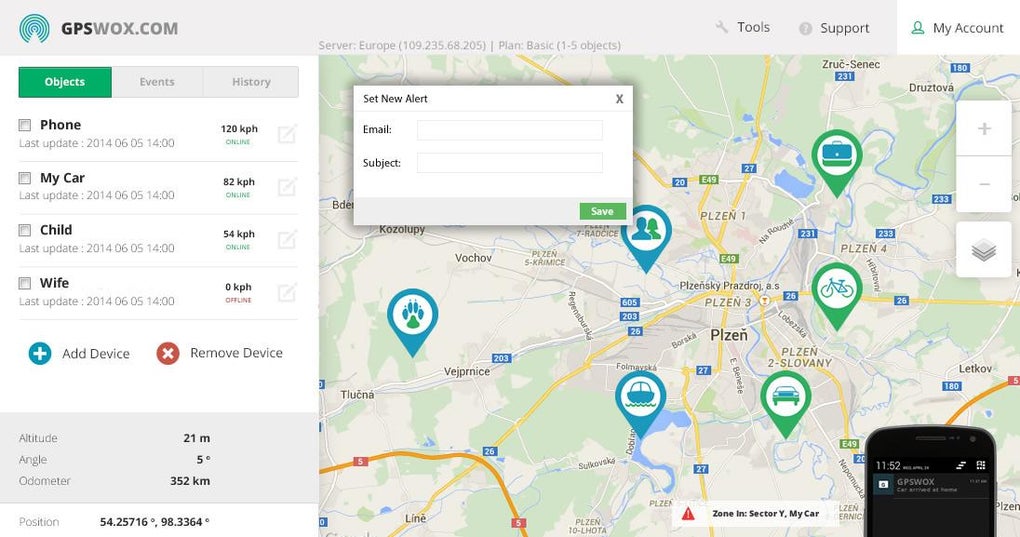This detailed image from the GPSWOX website showcases a comprehensive map, possibly of a European location, as indicated by the foreign-sounding place names. On the right-hand side of the application interface, several tabs are visible, including "Objects," "Events," and "History," with the "Objects" tab currently selected, highlighted by a green box. Further details under this tab reveal tracked items such as "phone," "my car," "child," and "wife," each displaying their respective speeds in kilometers per hour—120 km/h for the phone, 82 km/h for the car, 54 km/h for the child, and 0 km/h (offline) for the wife. Additionally, there are options to add a new device, marked by a plus sign, or remove a device, indicated by a red X in a box. A popped-up dialog box labeled "Set New Alert" includes fields for "email" and "subject," indicating functionality for customizing alerts.